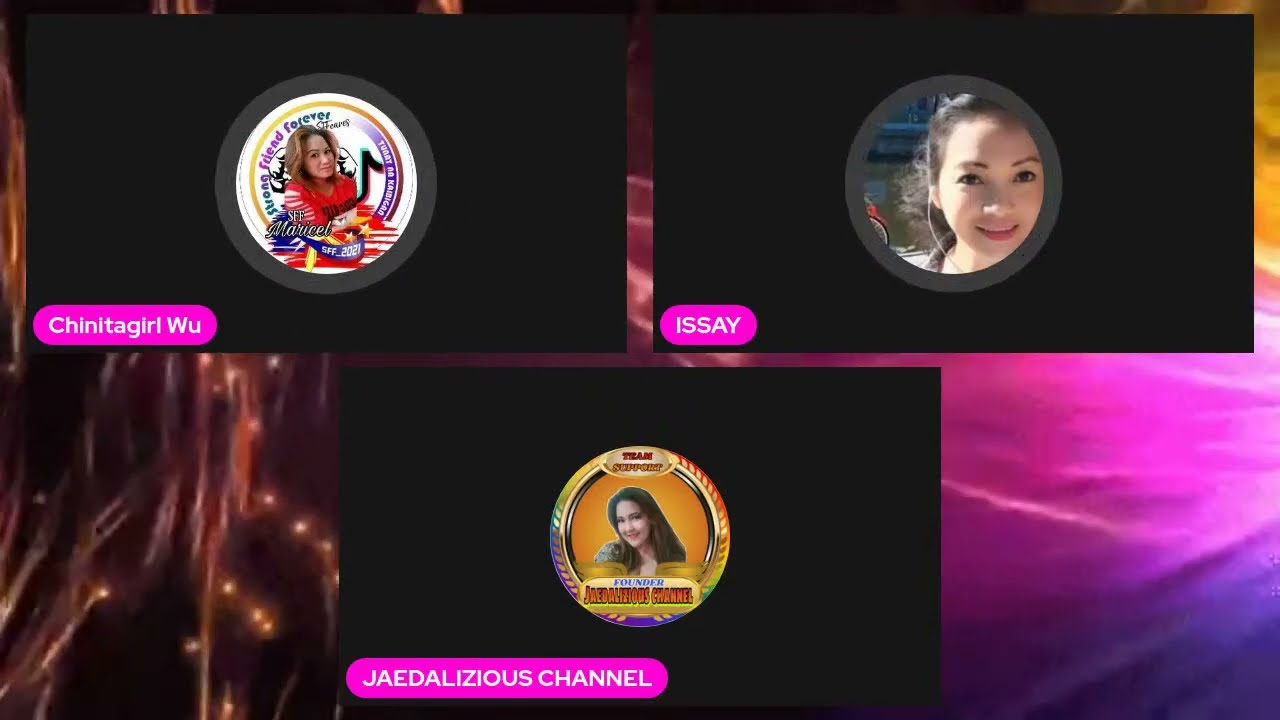The image depicts a vibrant digital interface with a background swirling with hues of pink, purple, white, black, and orange. Featured prominently are three black rectangles, each containing a circular portrait of an Asian woman, giving the layout a structured yet visually dynamic appearance.

In the top left corner, the black rectangle contains the text "Chinita Girl Woo" written in white on a pink text box. The portrait within shows a woman with light brown, shoulder-length hair wearing a red shirt, set against a backdrop featuring various logos.

The top right rectangle, labeled "Issay," also in white on a pink text box, displays a close-up of a smiling woman with dark hair tied back in a ponytail.

Centered below these two, the third black rectangle is labeled "Jadalicious Channel" in similar white text on a pink background. Within this rectangle is a circular portrait of a woman with long, medium brown hair, who is smiling and slightly leaning to the left, framed by a yellow circle.

Overall, the layout and the use of colors create an energetic and engaging visual that suggests a personal webpage or a YouTube channel interface.